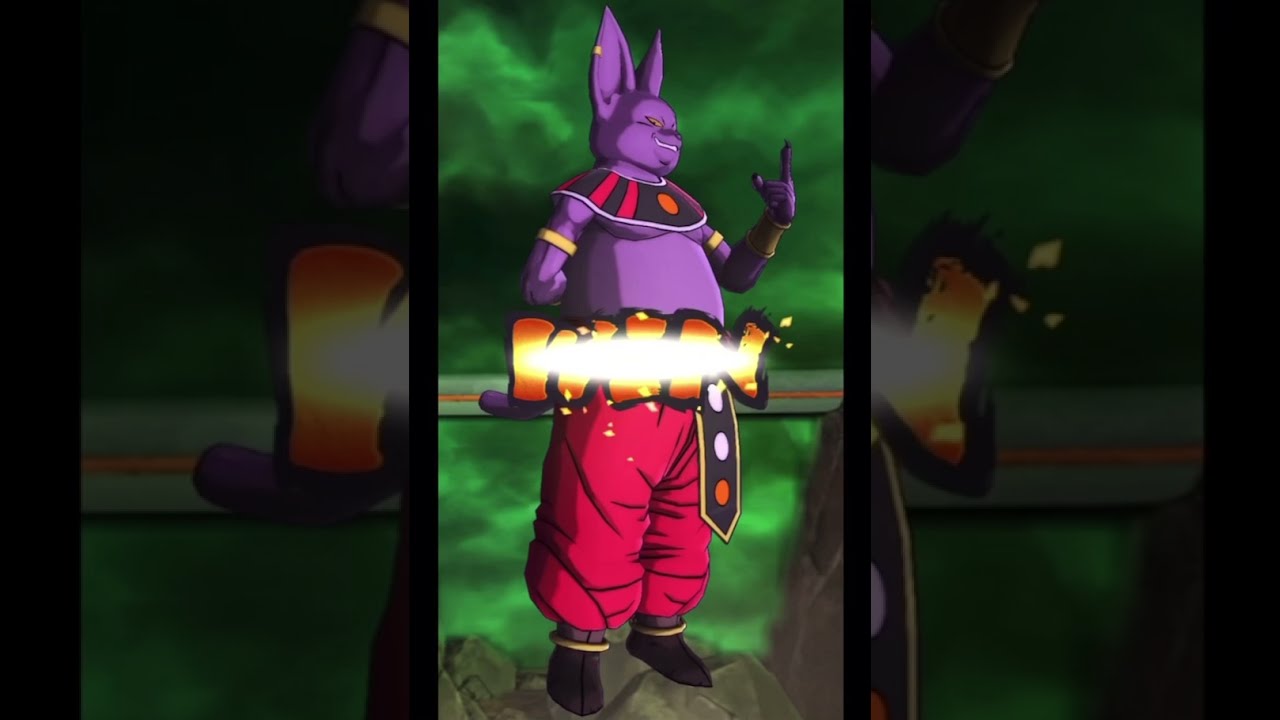The image depicts a vibrant, possibly video game or animated character with striking features. Centered against a green foggy background and rocky terrain, the character, resembling a tall and hefty Easter Bunny or alien fox, stands triumphantly. This purple-skinned being has two large, upright, pointy ears adorned with an earring. With yellow eyes and a broad smile, it conveys confidence. The character is shirtless, revealing a sash around its neck and shoulders, and is dressed in long red sweatpants and black shoes. Notably, it is gesturing proudly with its left arm raised, index finger pointed skyward. Dominating the foreground, bold letters spell "WIN" in orange and yellow, illuminated by a bright stripe, emphasizing the character’s victorious stance.